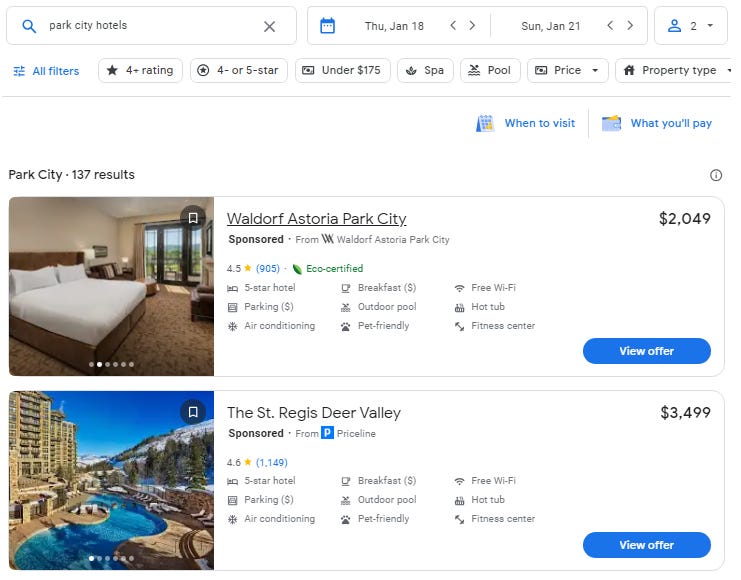Screenshot of a hotel booking website for Park City, showing results for a stay from Thursday, January 18th through Sunday, January 21st for two people. The filters are set to show hotels with a four to five-star rating under $175 per night, with amenities such as a spa and pool. The page displays 137 results, with an option to toggle property type. 

Visible are two specific hotel options:

1. **Waldorf Astoria Park City** (Sponsored by Waldorf Astoria Park City)
   - Price: $2,049 for the specified stay
   - Star Rating: 4.5 stars
   - Reviews: 9,105
   - Certification: Eco-certified
   - Classification: Five-star hotel
   - Amenities: Paid parking, air conditioning, paid breakfast, outdoor pool, pet-friendly, free Wi-Fi, hot tub, and fitness center.
   - Booking Option: A blue "View Offer" button is available for more details.
   - Accompanied by a photo of the hotel.

2. **The St. Regis Deer Valley** (Sponsored by Priceline)
   - Price: $3,499 for the specified stay
   - Star Rating: 4.6 stars
   - Reviews: 1,149
   - Classification: Five-star hotel
   - Amenities: Paid parking
  
To the right, there are links for "When to Visit" and "What You'll Pay" offering additional information to potential bookers.